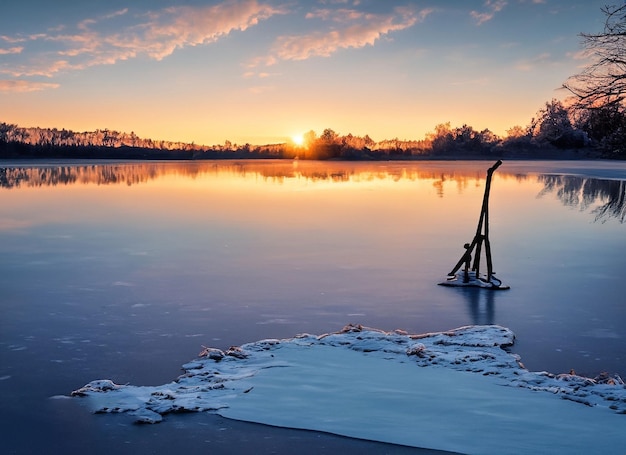This photograph captures a serene winter scene of a partially frozen lake, accented by a vivid sunrise or sunset just above the horizon. In the foreground, a snow-covered bank juts out into the lake, its pristine white surface contrasting with the icy water. Scattered on the lake's surface, a small wooden structure resembling a triangular frame or teepee made of sticks stands out, hinting at the possibility of ice fishing. The distant shore is lined with barren trees of varying heights, silhouetted against an orange and blue sky. The reflection of the reddish clouds on the lake's surface enhances the tranquil yet cold ambiance of the scene. Tree branches from the right side of the frame subtly intrude, adding an additional layer of depth to this picturesque winter landscape.